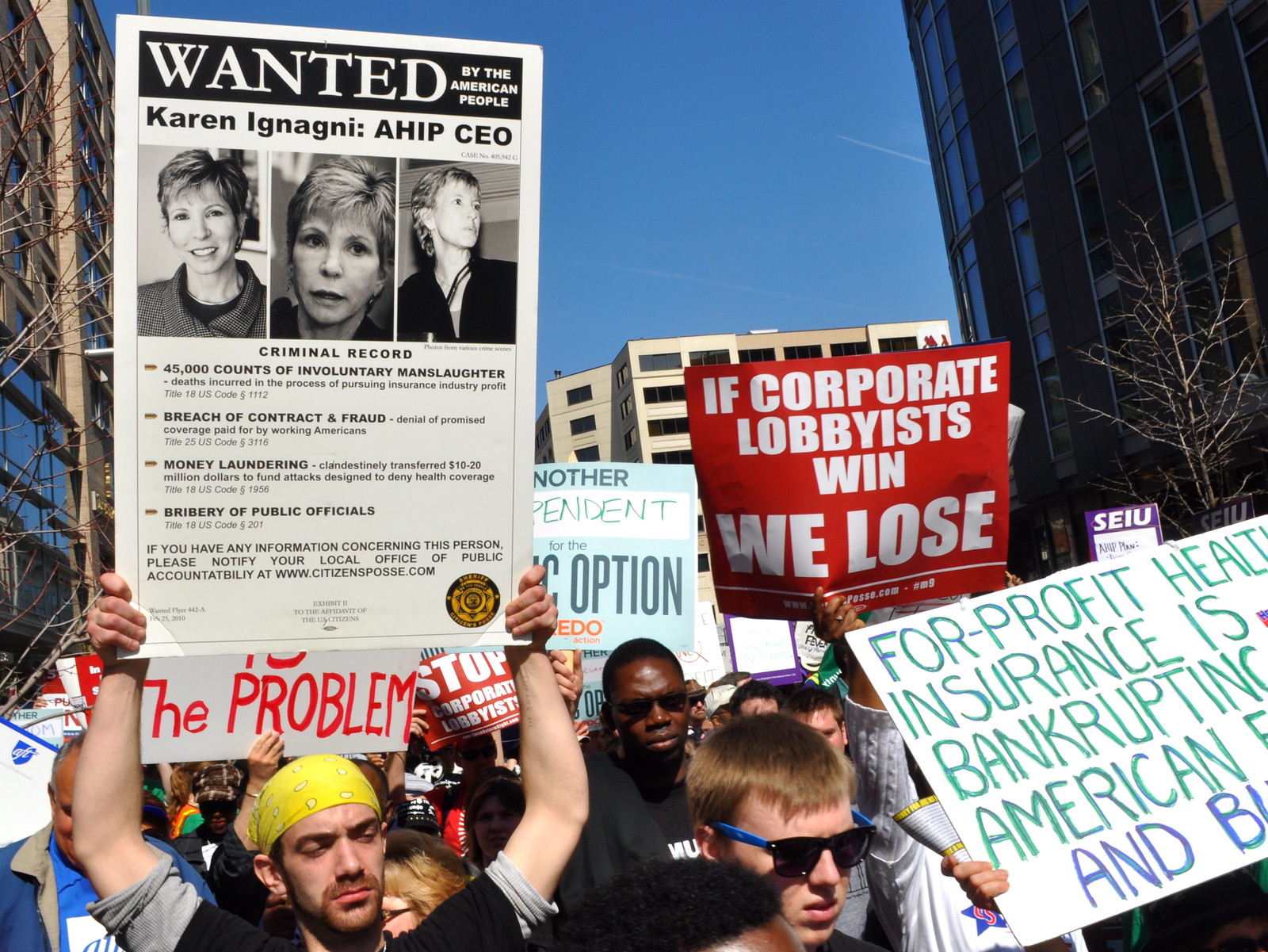In this full-color photograph taken on a sunny day with a bright blue, cloudless sky, a large outdoor protest is captured in an urban setting. The scene shows a diverse group of predominantly male protesters, situated in front of several tall office buildings that frame the background—a brown building on the left, a white building in the center, and another brown building on the right. The crowd, seen mostly from the torso up, holds a variety of hand-printed and professionally printed signs. 

Prominently on the left, a white man wearing a yellow bandana and a short-sleeved black shirt raises a white sign above his head. This sign is styled as a wanted poster and reads: "Wanted by the American People: Karen Ignagni, AHIP CEO," accompanied by three pictures of her and a list of alleged criminal charges, including "450,000 counts of involuntary manslaughter, deaths incurred in the process of pursuing insurance industry profit." 

To the right, a noticeable red sign declares, "If corporate lobbyists win, we lose." There's also a partially visible white sign on the far right, stating "for-profit health insurance is bankrupting American families and business," though the ends of the sign are cut off. The image evokes a strong sense of activism reminiscent of an Occupy Wall Street protest, with the protesters' determined expressions and the varied messages depicted on their signs.